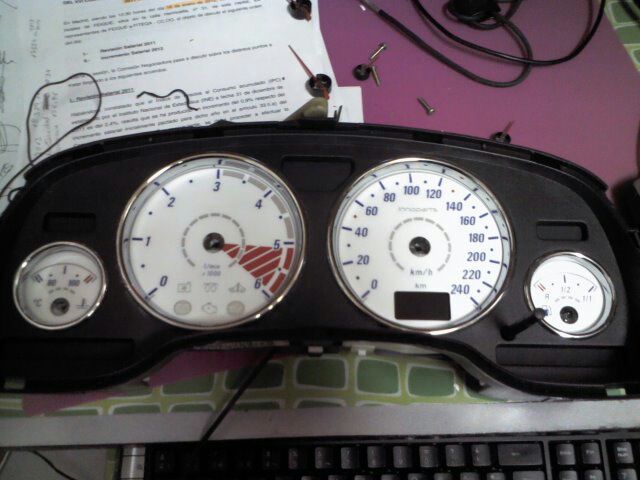In the photograph, a small, sophisticated dashboard featuring four distinct dials is prominently displayed. Each dial seems to measure different parameters, most likely pressures. 

On the left-hand side, the first dial is small with a white background and fine red and black lettering, indicating varying pressure levels. The second dial is noticeably larger, with a white background, black numbering from 0 to 6, and a small red cone between the 5 and 6, probably signaling critical levels. The third dial, also with a white background, has black numbers ranging from 0 to 240 in increments of 20, laid out in a circular fashion. The fourth dial mirrors the first, being small and likely another pressure gauge.

These four dials are set on a sleek, black-silver dashboard. Below this, in the lower section of the photograph, the top portion of a black desktop keyboard is visible. 

In the top left-hand corner, a sheet of paper with extensive printed text and some portions highlighted in orange is seen. In the top right corner, there are several loose screws and bits of cabling scattered on the table. The table itself is a striking purplish violet color.

The image centers on the detailed dials mounted on the dashboard, while also capturing the surrounding work environment elements such as the keyboard, paper, and table.